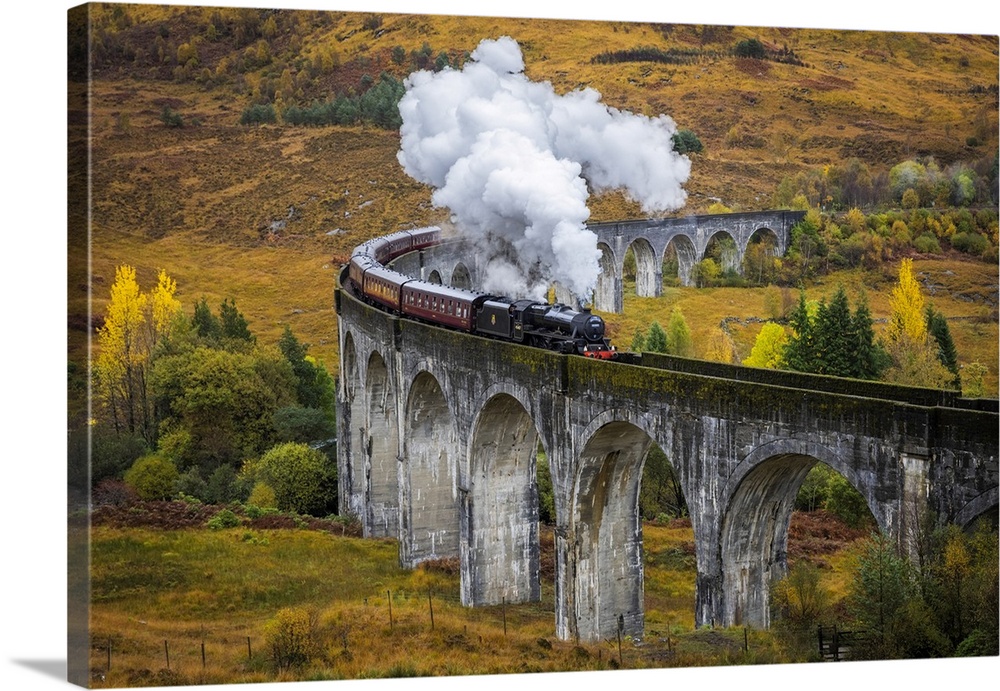The image portrays a steam train, with a single engine and multiple passenger cars, crossing a high, weathered stone bridge with archways. The bridge, likely 60 to 70 feet above the ground, is famous for its curved design, which the train is navigating as it emits heavy plumes of white and gray steam. The scene is set against a backdrop featuring a barren, rocky terrain, with the distant side of a mountain, and interspersed tree-lined areas that show signs of fall with changing leaves. Below the archways of the bridge, various bushes and trees add to the serene beauty of the landscape. The entire composition might be a painting, giving an impression of a secluded area untouched by human habitation.